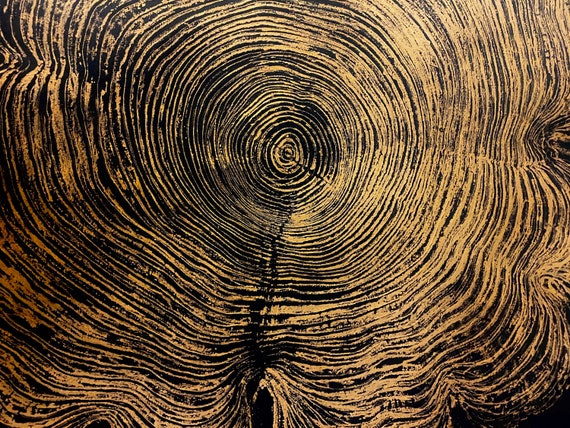This image is an abstract illustration reminiscent of a tree stump's cross-section. It features numerous concentric rings that evoke the natural age lines of a tree trunk. The rings start more circular and regular at the center, gradually becoming irregular and wavy as they move outward, creating a distinctly ruffled edge. Predominantly, the rings are rendered in shades of tanny brown and a pale goldish yellow, interspersed with striking black lines that highlight the natural wood grain texture. The overall palette gives the illustration a lifelike, naturalistic feel akin to an aged tree trunk. Background elements hint at a darker, perhaps purplish brown shade, adding depth and contrast to the intricate ring patterns. Some cracks and inclusions can be spotted, further enhancing the realistic portrayal of tree rings. An intriguing detail is a central bullseye-like circle, possibly indicating an arrow stuck in the middle, which adds an unexpected focal point to this richly detailed and textured artwork.